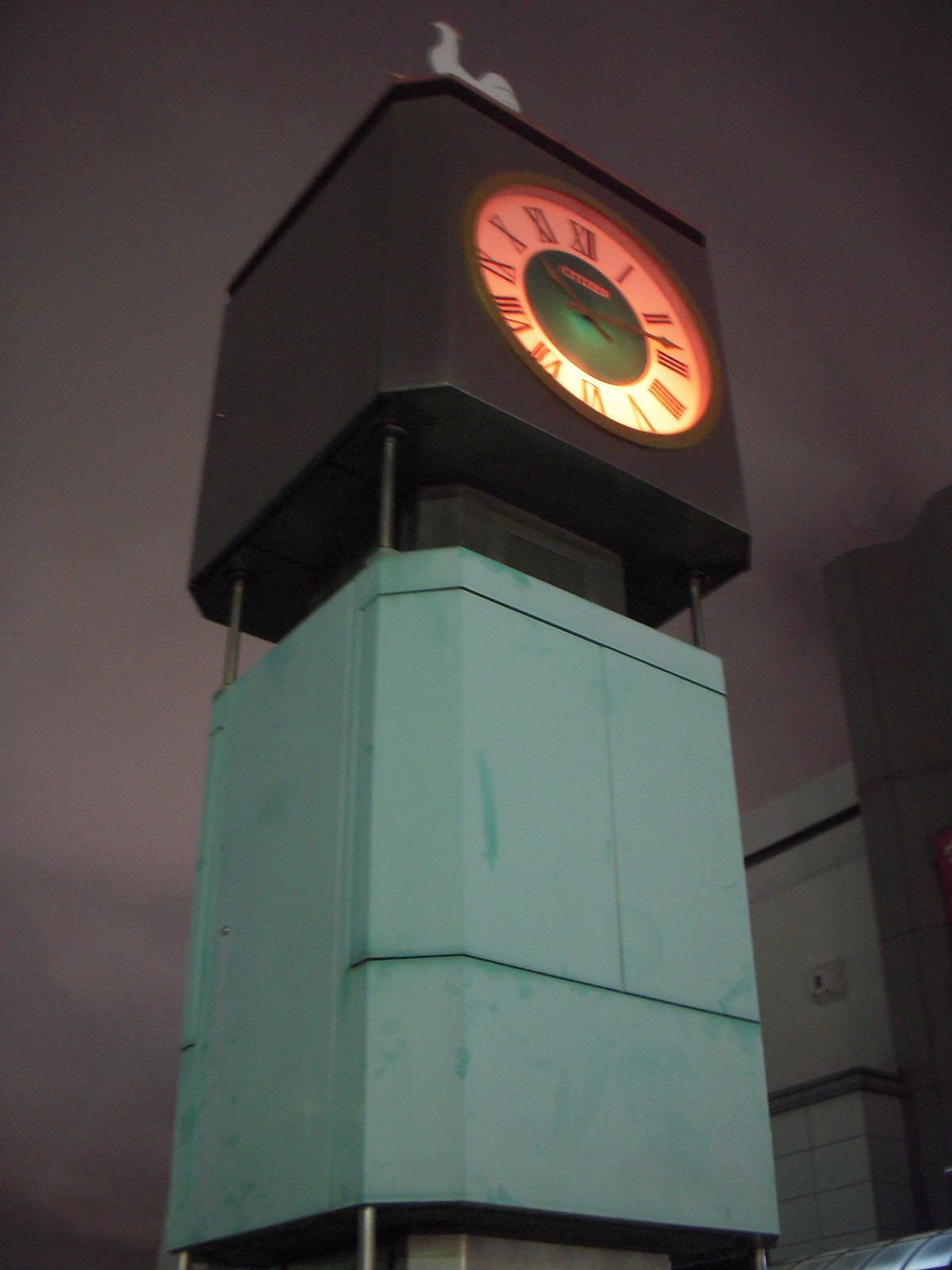This image captures a striking clock tower, characterized by its unique and somewhat simplistic design. The tower features a rectangular, greenish metal base at the bottom, transitioning to a dark brown or black square section at the top that houses the clock itself. The clockface is circular, lit with a yellowish-red glow, and features Roman numerals in black around a white circumference. The green center of the clock adds a distinct color contrast against the darker hues. The clock shows the time as approximately 9:14 or quarter past 10, with its hands in a dark brown color. At the very top of the tower, there is a white rooster or chicken figure, possibly serving as a weather vane or decorative element, with discernible feathers and tail pointing upward. The backdrop reveals a dark, cloudy sky, adding a moody atmosphere to the scene. In the right-hand side of the image, two buildings are partially visible; one is white with a tiled base and a square feature that resembles an electrical outlet, and the other is black, with only a corner showing.